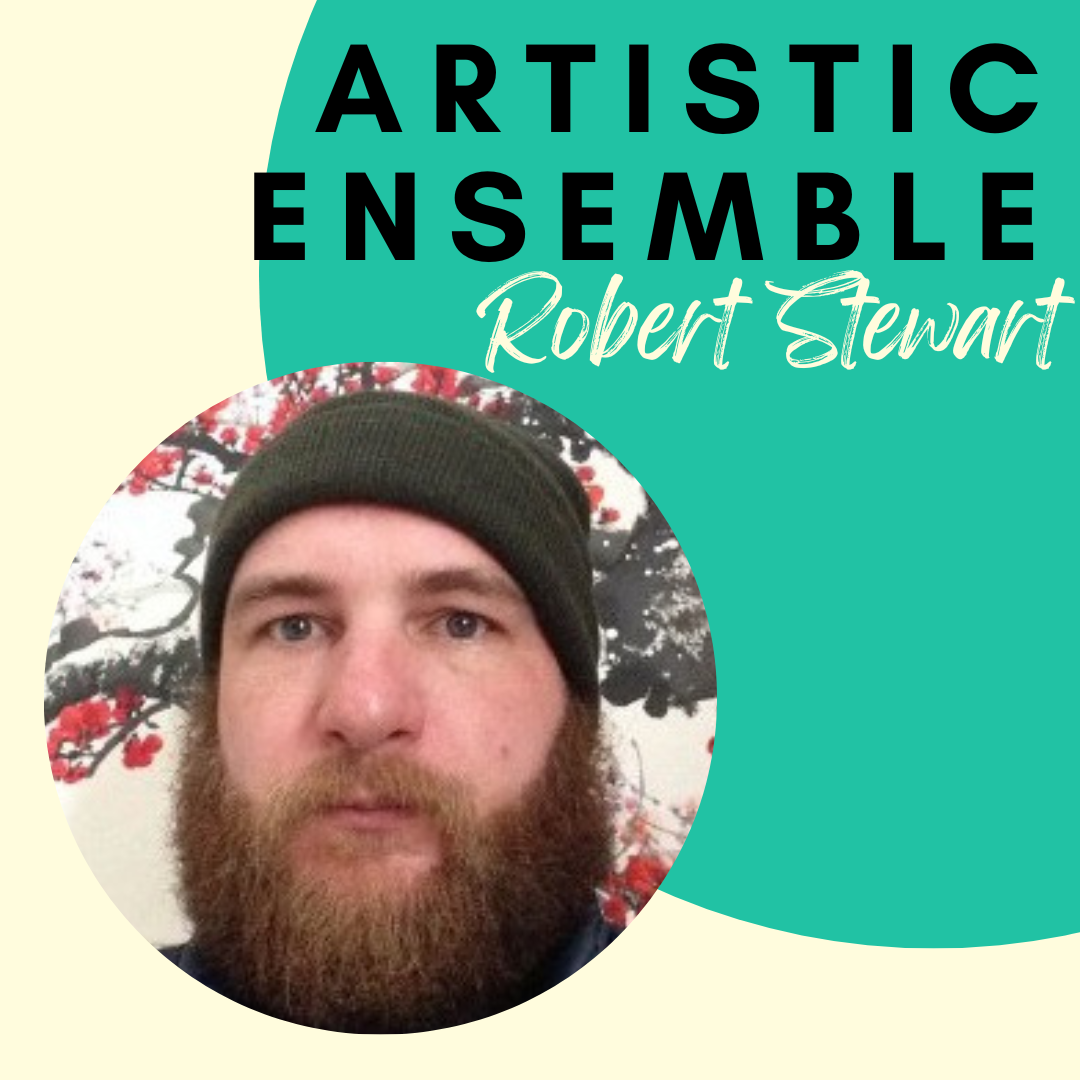This is an image, possibly a promotional cover, featuring a man named Robert Stewart. His face is prominently displayed in a circle in the bottom right corner. He is a white man with a thick, reddish-brown beard and mustache, and he appears to have brown eyes, though the image quality makes it slightly difficult to confirm. He is wearing a dark, toboggan-style knit cap, possibly blue or greenish-black, and a dark sweater.

The background of the image is primarily manila yellow with a multicolored section that includes a painting of a tree in red, white, and black hues. In the top right corner, there is a partial circle with black block text that reads "Artistic Ensemble," and underneath, in a more curvy white font, it says "Robert Stewart." The overall design suggests that this image serves as an advertisement or a book cover highlighting Robert Stewart as an artist.